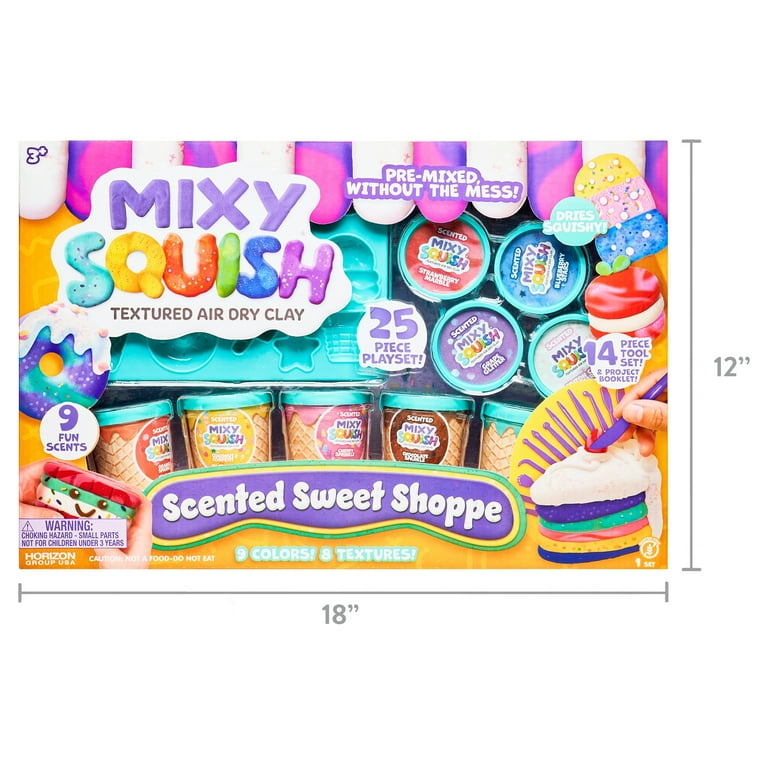The image showcases a product listing for a vibrant and colorful box titled "Mixy Squish Textured Air-Dry Clay - Scented Sweet Shop." The box promises pre-mixed clay that avoids the mess, featuring nine fun scents, nine colors, and eight textures. There is a clear plastic window on the front of the box revealing tubs of clay in various shades, including red, yellow, pink, brown, and green. The box prominently displays images of potential creations like ice cream cones, cookies, and cakes, emphasizing its pastry and bakery-themed items. Textures and color combinations allow kids to craft detailed and realistic-looking sweets. The product is marketed as a 25-piece playset that includes molds for shaping the clay into forms such as stars. Measuring 12 inches tall and 18 inches long, the product appears to float in an empty white space, making it the focal point of the image. Important safety information includes a warning about small parts being a choking hazard for children under three, a caution that the product is not food, and the manufacturer's name, Horizon Group, located in the lower left corner.